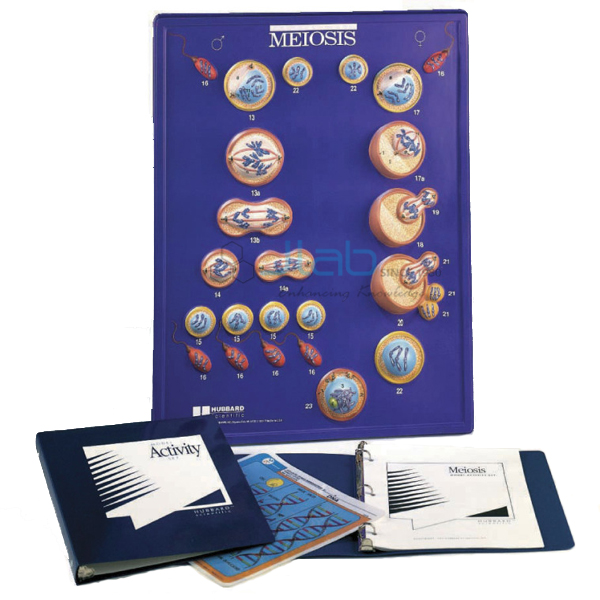The image depicts a detailed educational setup focused on the process of meiosis. Dominating the top portion is a large, blue-background chart with "MEIOSIS" emblazoned in bold, white, all-caps letters. The chart is divided into male and female sections, marked by their respective gender symbols. It illustrates the stages of meiosis with a sequence of images: starting with what appear to be sperm cells, followed by various stages represented by circles, peanut shapes, and larger circles. Each image is numbered for reference.

Beneath this vivid chart, a black binder labeled "activity" in black letters rests closed, while another binder positioned slightly below to the right is open, displaying white pages. The first visible page in the open binder also bears the title "meiosis." Between the two binders lies a loose sheet of blue paper adorned with DNA diagrams. The chart and binders suggest a comprehensive educational kit from Hubbard Scientific, aimed at enhancing laboratory knowledge on cellular reproduction.